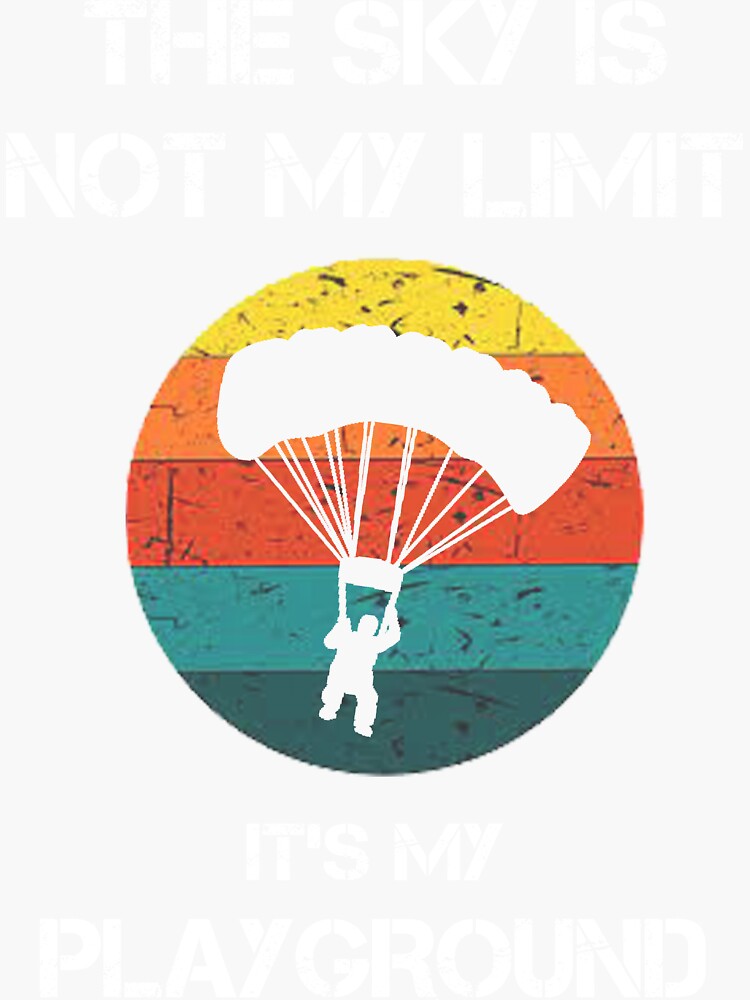The image is a motivational poster featuring a central circular design with a multicolored background. The background is composed of five horizontal stripes in yellow, orange, red, light blue, and dark blue. In the center of this circle, a parachutist is depicted as a white silhouette, holding onto the side straps of a parachute. The parachutist is shown flying towards the lower right, against the vibrant gradient of colors. Above the parachutist, in large white text with a slightly edgy, smudged look, the motivational phrase reads, "The sky is not my limit, it's my playground." The contrast of the text with the background may not be the best, adding a raw, artistic touch to the illustration. The overall image blends the thrill of adventure with a powerful motivational message, encouraging viewers to see the sky as a limitless playground.